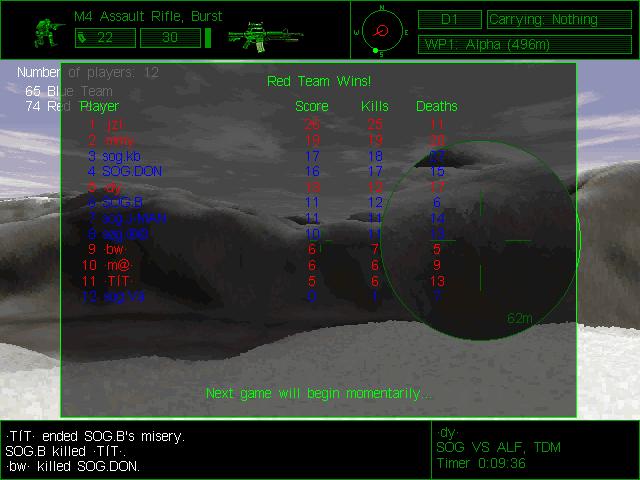This detailed caption synthesizes the common elements and emphasizes the repeated details:

This is a screenshot from a first-person shooter video game. In the foreground, a black opaque rectangular leaderboard displays the names and scores of 12 players, split between the blue team and the red team. The red team has won with a score of 75 to the blue team's 65, as indicated by green text reading "Red Team Wins." Each player's kills and deaths are listed in lime green, with notable scores including a player denoted by "Z" with 25 kills and 11 deaths, and others such as MMY with 19 kills and 20 deaths, and SOGKB with 18 kills and 22 deaths. At the bottom of the rectangle, highlighted in lime green, the notice "Next game begins momentarily" appears. The background features snowcapped grey mountains beneath a greyish-blue sky with white clouds and patches of snow at the base. Additional black text boxes on the left side provide game events, such as "TIT ended SOGB's misery" and "BW killed SOGDON," while the right side includes lime green text stating "DY SOG vs ALF" and "TDM timer 0.09..36." The colors in this screenshot are predominantly green, red, blue, grey, and black. The image also includes various in-game elements like names and scores indicative of a multiplayer game mode.